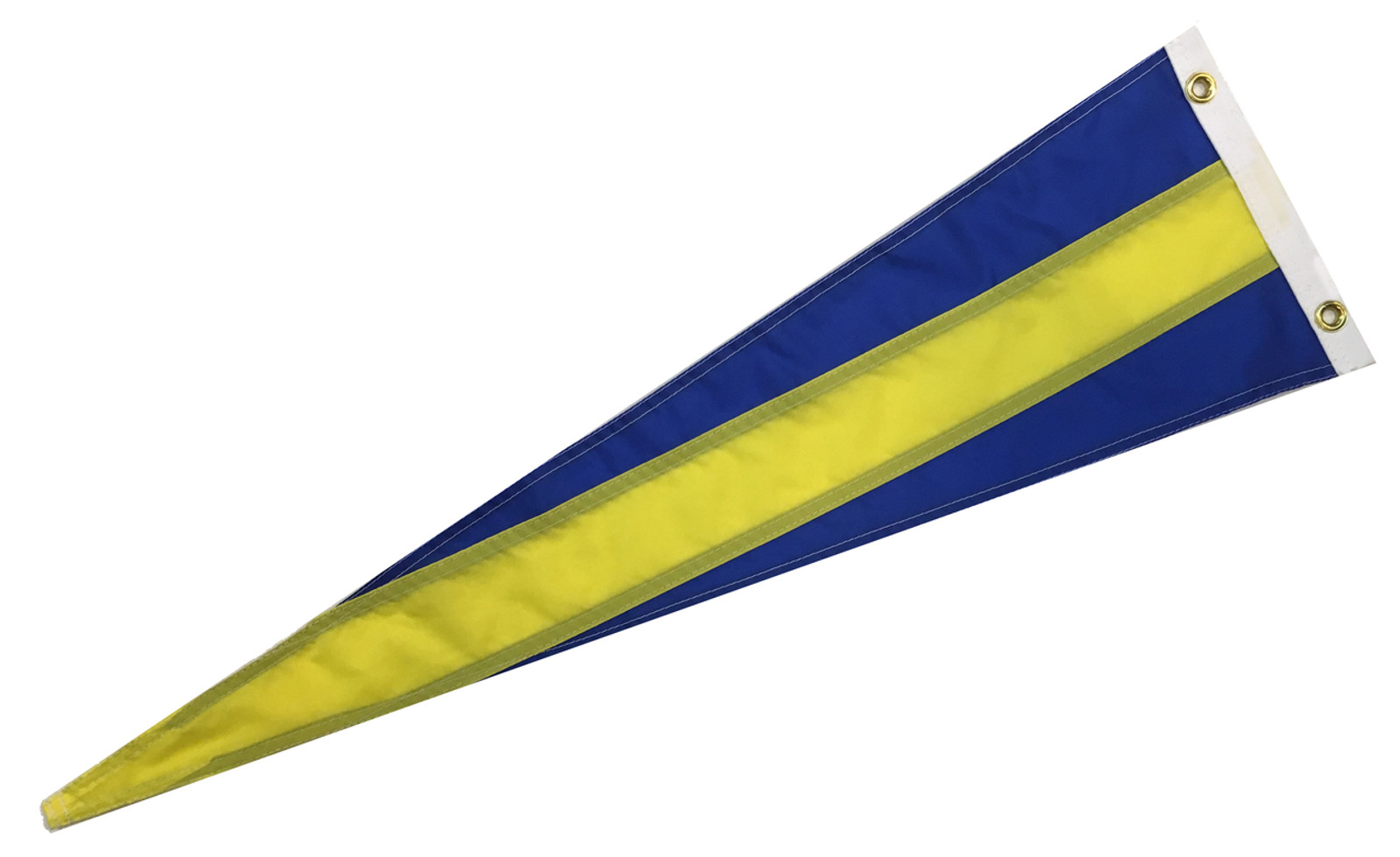This photograph captures a distinctive pennant flag set against a solid white background. The flag, which is elongated and triangular, appears to be exceptionally long and narrow. With an aspect ratio suggesting that the sides of the triangle are roughly five times the length of its base, the flag’s design is quite striking.

Toward the top of the triangle, the flag features two gold grommets on a thickened white strip for durability, where it can be hung. This white side is directed towards the upper right corner of the image, causing the triangle to descend to a point in the lower left corner.

The flag is divided into three horizontal stripes: the top and bottom thirds are a deep blue, while the center stripe is a darker yellow. Unusually, this yellow stripe extends all the way to the tip of the triangle, with the blue segments tapering off about three-quarters of the way down the flag. The overall design is simple yet bold, reminiscent of a college pennant flag, though it lacks any text or insignia.